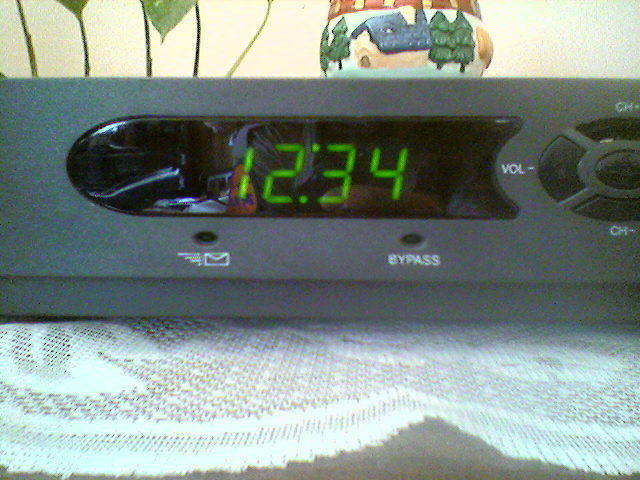The photograph features a bulky, dark silver and black cable box, situated on top of a white lace doily, with dark wood visible beneath it. The digital clock on the front of the cable box displays the time 12:34 in bright green. The device's front panel includes several buttons: "channel up," "channel down," and "volume down" in white font. The section under the clock also displays the word "bypass" in white, alongside a small black button. Adjacent to this are additional buttons marked with an envelope icon and some slash lines. Above the cable box sits a ceramic knick-knack depicting a white house with a blue roof and green trees. In the background, there are several green plant stems and a piece of colorful pottery with red, blue, green, and tan hues.